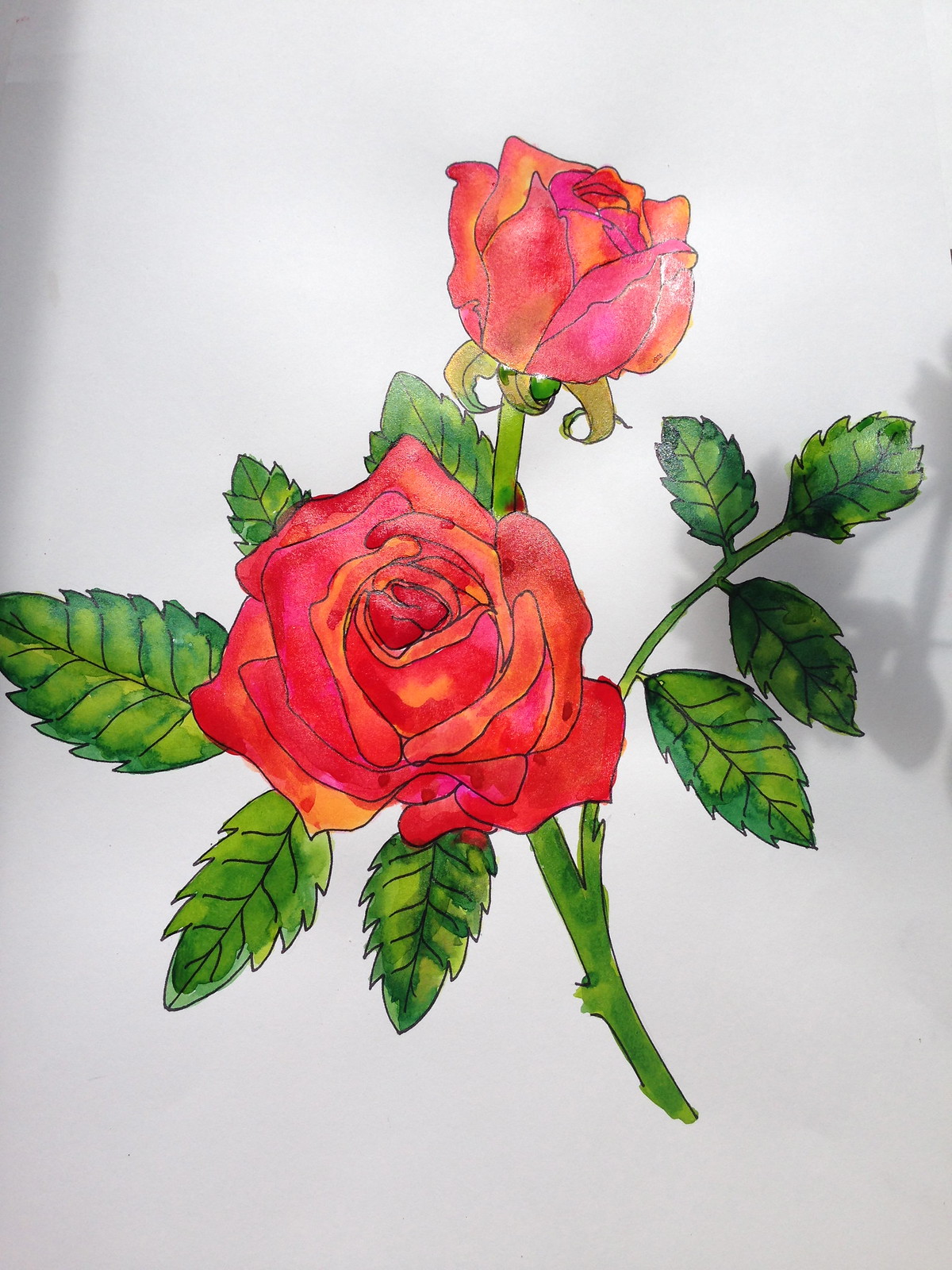The image showcases a detailed artwork featuring two exquisite red roses with numerous petals, positioned amidst a vivid green stem adorned with nine lush green leaves. The roses are placed such that one is centrally located while the other is higher up. The artwork is rendered on a pristine white background, which enhances the vibrancy of the colors. A subtle gray shadow of the artwork is visible on the right, adding depth to the otherwise plain background. Overall, the composition emphasizes the intricate beauty of the roses and leaves, with careful attention to detail evident in the lush petals and verdant foliage.